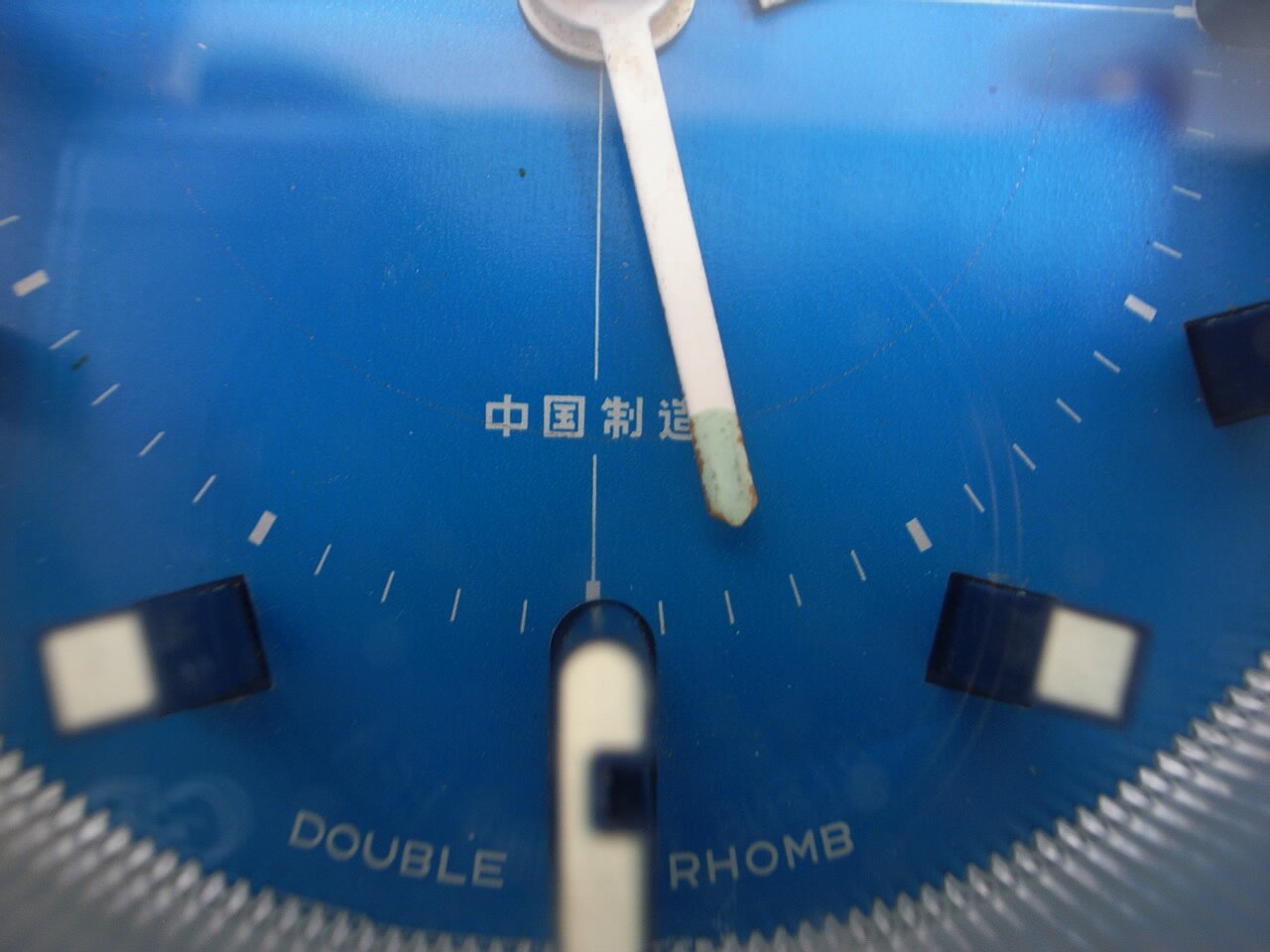This close-up image reveals the intricate details of a clock face, likely that of a wristwatch. The circular frame is a silver-gray metal, providing a sturdy border to the vibrant blue face. The clock does not feature conventional numbers; instead, it has white notches and square pegs to mark the hours, with bolder notches indicating the main hour points. A single watch hand, with a green-tinted tip that appears slightly stained, is visible near the bottom center.

The clock face includes several black and white accents, adding to the complexity of its design, though the image is slightly blurry around these elements due to the extreme close-up nature of the photo. Notable text at the bottom reads "double RHOMB" in white letters, and above this, there's writing in an Asian language, possibly Korean, Japanese, or Chinese. The clock also displays signs of wear and tear, hinting it is not new.

Given the angle and zoom level of the image, it's challenging to determine the clock's full appearance or even if it is part of a wristwatch, pocket watch, or wall clock.